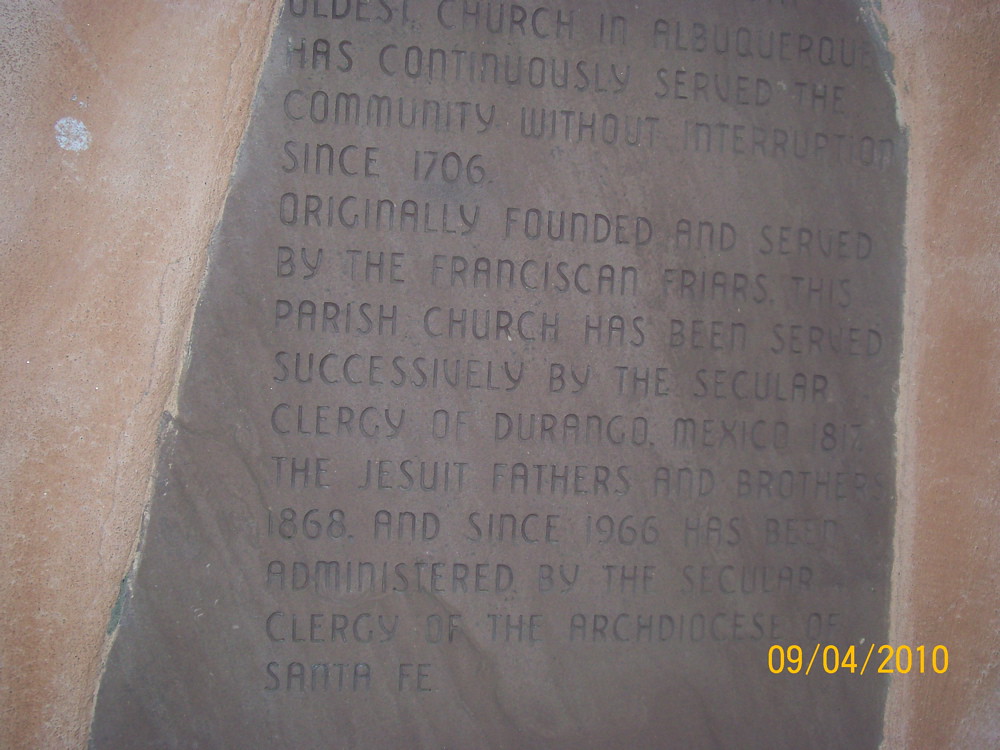The image showcases a stone plaque embedded in a larger, rugged rock formation that appears grayish-red with mild white patches. The plaque itself is a dark gray slate with carved, legible black lettering. The text commemorates the oldest church in Albuquerque, which has continuously served the community since 1706. Initially established and managed by Franciscan friars, the church later received the service of the secular clergy of Durango, Mexico in 1817, followed by the Jesuit fathers and brothers in 1868. Since 1966, it has been administered by the secular clergy of the Archdiocese of Santa Fe. In the bottom right corner of the plaque, the date '09/04/2010' is inscribed in gold-yellow text, reminiscent of a timestamp from a digital camcorder.